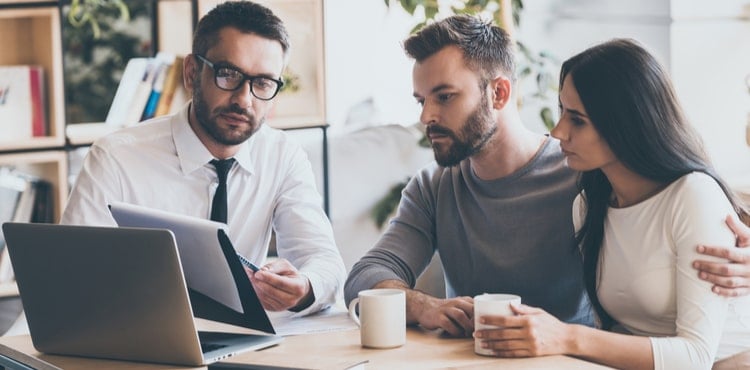This color photograph, shot in landscape orientation, depicts a detailed scene of a business meeting between three individuals sitting at a light wooden table. On the left, a man with short dark hair, dark-framed glasses, a mustache, and a beard is dressed in a white collared shirt paired with a black tie. He is holding a pen in his left hand, which he uses to point at a clipboard in front of him, suggesting he is presenting or explaining something. Just behind the clipboard, an open laptop is positioned, although its screen is not visible to the viewer.

In the middle of the photograph, a young man with a similar short dark hair and beard is clad in a long-sleeved gray shirt. He appears to be focused on the clipboard, listening intently. This man has his right arm comfortably draped around the shoulders of the woman sitting to his right. In front of him, a white coffee cup with its handle pointing left is placed on the table.

The woman on the far right has long, straight, dark hair cascading down her back and is dressed in a white long-sleeved top. She appears deeply engaged, her attention fixed on the clipboard as well. Lightly holding a second white coffee mug with her left hand, her body language mirrors a sense of involvement in the discussion.

Background elements, slightly blurred, include shelves stocked with books or documents and some greenery, adding to the ambiance of a professional office. The overall colors in the photograph are muted, enhancing the serious and contemplative atmosphere of the meeting. The image effectively captures a consultant, possibly a broker, advisor, or insurance agent, presenting critical information to a couple, as indicated by the man’s arm wrapped around the woman.